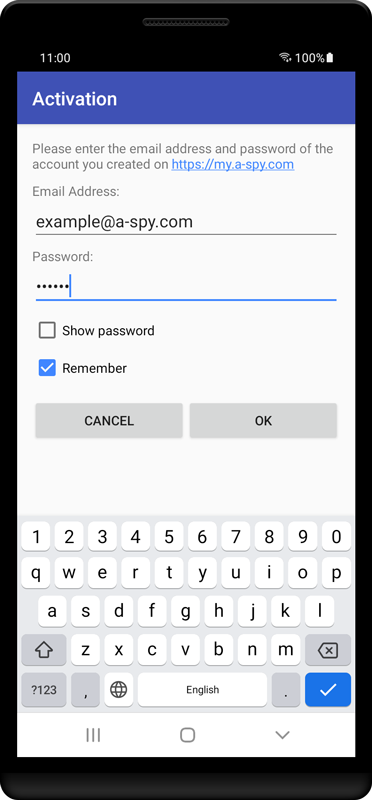The image depicts the screen of a cell phone, showcasing a detailed account activation page. The phone has a standard black border surrounding the screen. 

At the top left corner of the screen, the time is displayed as 11 o'clock. On the opposite side, the top right corner indicates a 100% battery life accompanied by a battery icon. 

Directly below this information, a prominent blue banner spans the width of the screen, with "Activation" written in large white text. Below this banner, the text prompts the user to "Please enter the email address and password of the account you created on https://my.a-spy.com." An email address, "example@a-spy.com," is already filled in.

Underneath the email field is the word "Password," followed by six asterisks representing the hidden password. Below the password field are two checkbox options. The first box, which is not checked, has the label "Show password." The second box, which has a blue background and a white checkmark, is labeled "Remember."

Further down, there are two buttons with gray backgrounds. The button on the left reads "Cancel," while the button on the right reads "OK." 

At the bottom of the screen is an alphanumeric keyboard. The top row displays numbers 1 through 0, followed by the standard QWERTY keyboard layout. 

Finally, three icons are displayed at the bottom of the page: three vertical lines, a square, and a downward-pointing arrow.